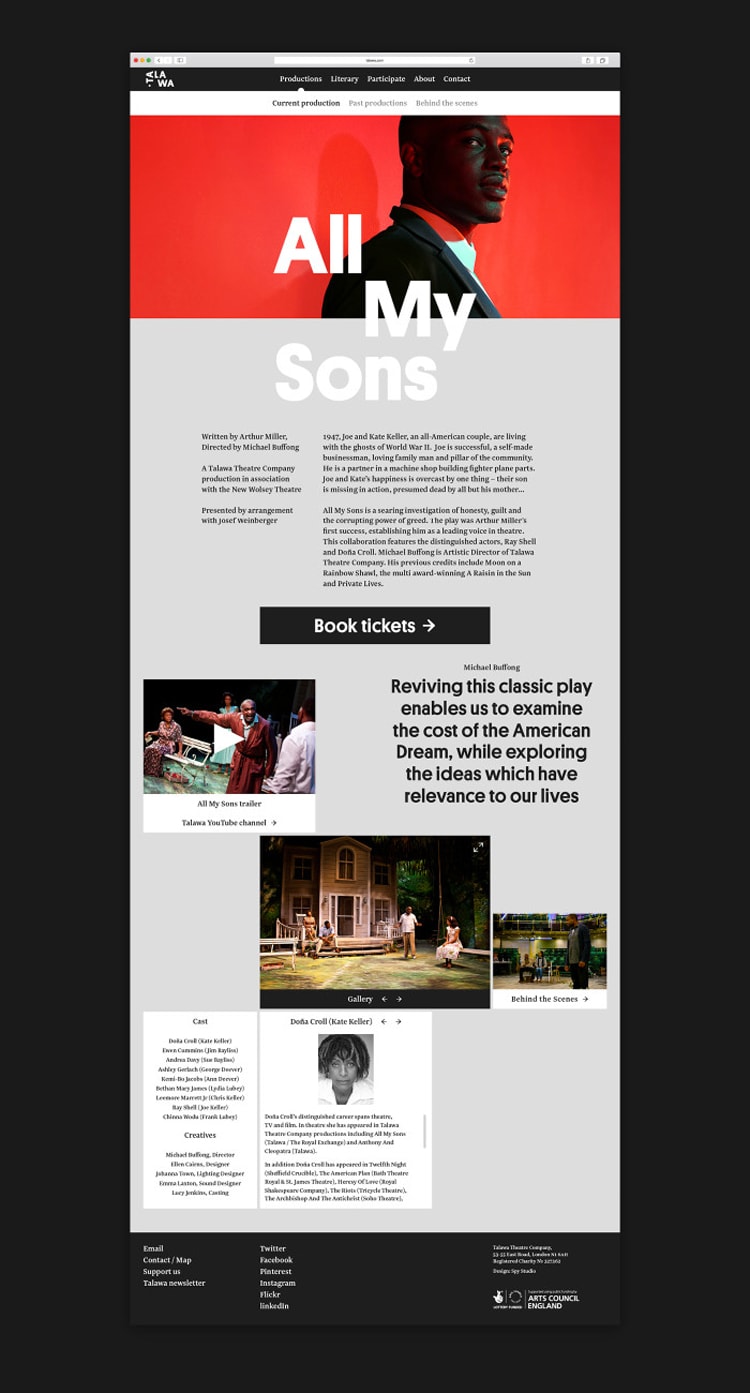This screenshot displays a web page from the TALAWA Theatre Company. At the top of the page, navigation options include "Productions," "Literary," "Participate," "About," and "Contact." Under "Productions," users can access sections for "Current Production," "Past Productions," and "Behind the Scenes."

The featured production on this page is "All My Sons," written by Arthur Miller and directed by Michael Buffong. This TALAWA Theatre Company production is presented in association with the New Wolsey Theatre and arranged by Joseph Weinberger.

The play is set in 1947 and centers around Joe and Kate Keller, an all-American couple grappling with the lingering effects of World War II. Joe Keller is portrayed as a successful self-made businessman, a loving family man, and a pillar of the community, involved in a machine shop that manufactures fighter plane parts. Despite their apparent success, Joe and Kate’s happiness is overshadowed by the haunting absence of their son, who is missing in action and presumed dead by everyone except Kate.

"All My Sons" is described as a powerful examination of honesty, guilt, and the corrupting influence of greed. Arthur Miller's first major success, the play established him as a leading voice in theatre. The production features esteemed actors Ray Schell and Donna Kroll.

The page includes images and videos that showcase various scenes from the play, the cast, and behind-the-scenes content. Michael Buffong serves as the artistic director for TALAWA Theatre Company.